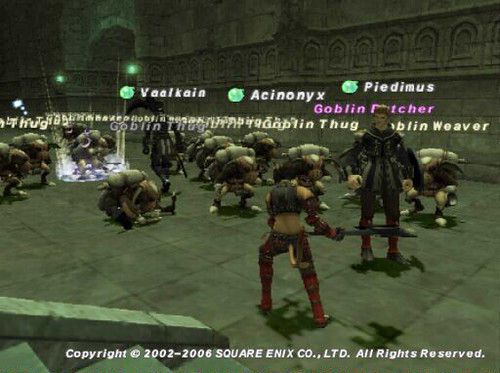Screenshot from a video game displays a scene set inside what appears to be a stone-walled castle, casting a greenish hue over the environment. At the bottom of the screen, the copyright notice "2002-2006 Square Enix Co. Ltd. All Rights Reserved." is clearly visible in white text.

The focus of the image is on a taller humanoid character standing in the foreground, facing the viewer. Surrounding him are seven smaller characters that resemble minotaurs, each carrying distinct backpacks. These minotaur-like figures are dispersed around the larger character in what appears to be a semi-circle.

Another character, different from both the humanoid and minotaur-like figures, stands directly opposite the tall humanoid. This character is equipped with red boots and holds a weapon, suggesting a potential confrontation. The stone walls and floor confirm the indoor castle setting, with subtle lighting enhancing the greenish atmosphere of the scene.